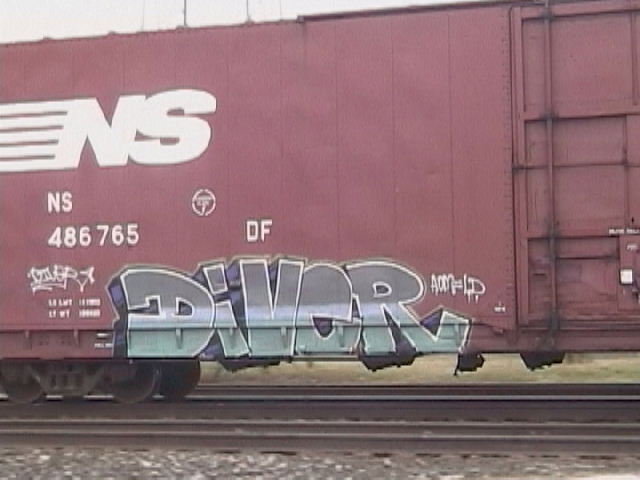This close-up photograph captures approximately two-thirds of a moving railroad car, which is painted a faded red typical of many railroad cars. The car sits on gray railroad tracks nestled in gravel. Prominently featured in the upper left section of the car is a logo accompanied by the letters "NS" printed beneath it, followed by the numbers "486765." To the right of this identification, the letters "DF" are inscribed. Adorning the lower part of the car is graffiti that reads "D-I-V-E-R" in green, while additional, smaller graffiti, which is difficult to decipher, appears on both sides. To the right, part of a sliding door is visible, contributing to the detailed industrial aesthetic of the image.